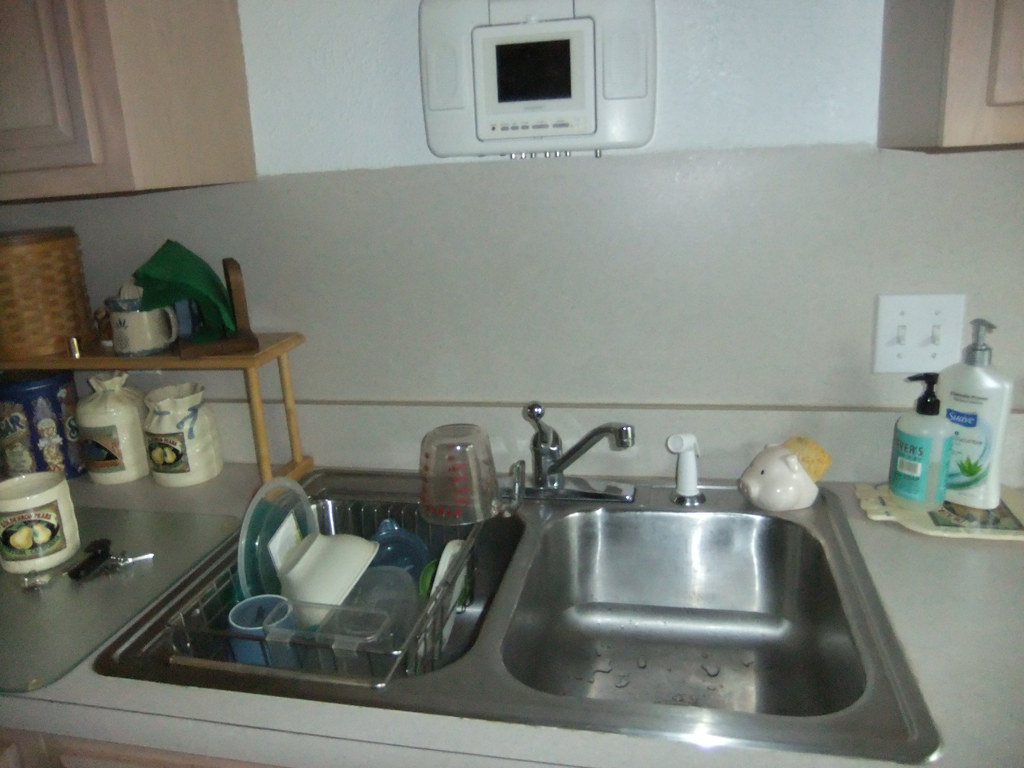The image showcases a sizable, stainless steel kitchen sink featuring two spacious tubs and a single-handle faucet. One of the tubs contains an in-sink drying rack with several dishes stacked upside down. A measuring cup precariously balances on the edge of the tub by the faucet. The kitchen presents a neat and organized appearance. 

On the countertop to the right of the sink, there's a trivet holding a bottle of Suave hand cream and a bottle of liquid soap. A decorative pig image, holding a sponge, adds a whimsical touch to the space. To the left of the sink, several matching containers of varying sizes are neatly arranged, likely filled with common kitchen staples like flour, sugar, and brown sugar. These containers are situated below a small wooden shelf that supports a wicker basket holding a coffee cup and a green napkin.

A glass cutting board is positioned to the left of the sink. Placed upon it are another coffee cup and a set of keys. Above the sink, an electronic device, possibly an alarm or stereo system, is mounted on the wall.